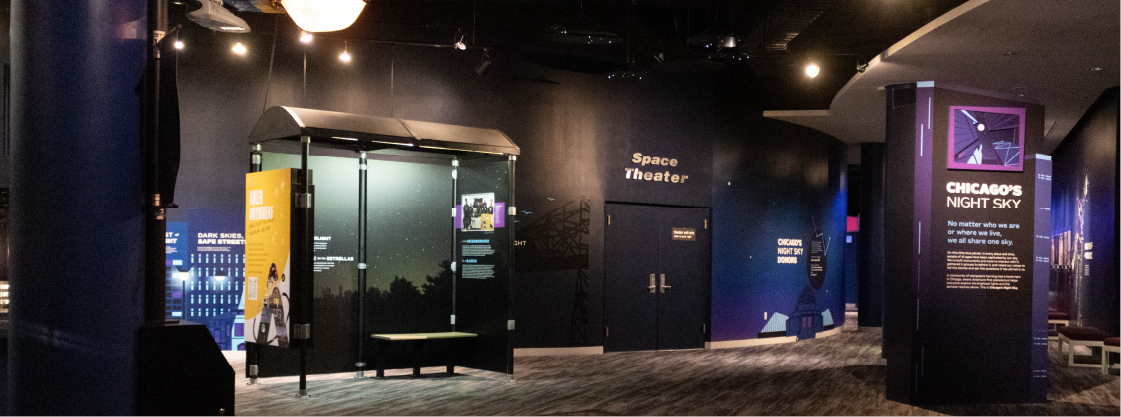The photograph captures the interior of a theater or planetarium with a dark, atmospheric setting illuminated by various ceiling lights. At the center of the image, there's a bus stop structure with a bench in front of it and two posters on display. To the right of this structure, two dark double doors are visible. Above these doors, the words "Space Theater" are prominently displayed in white font. Moving further to the right, the scene reveals a hallway and a column adorned with a poster that reads "Chicago's Night Sky." Additionally, there's partly visible text saying, "no matter who we are or where we live, we all share one sky." The flooring features a thin carpet with grey and cream striations, and the walls of the theater are predominantly black, enhancing the dramatic ambiance of the space.